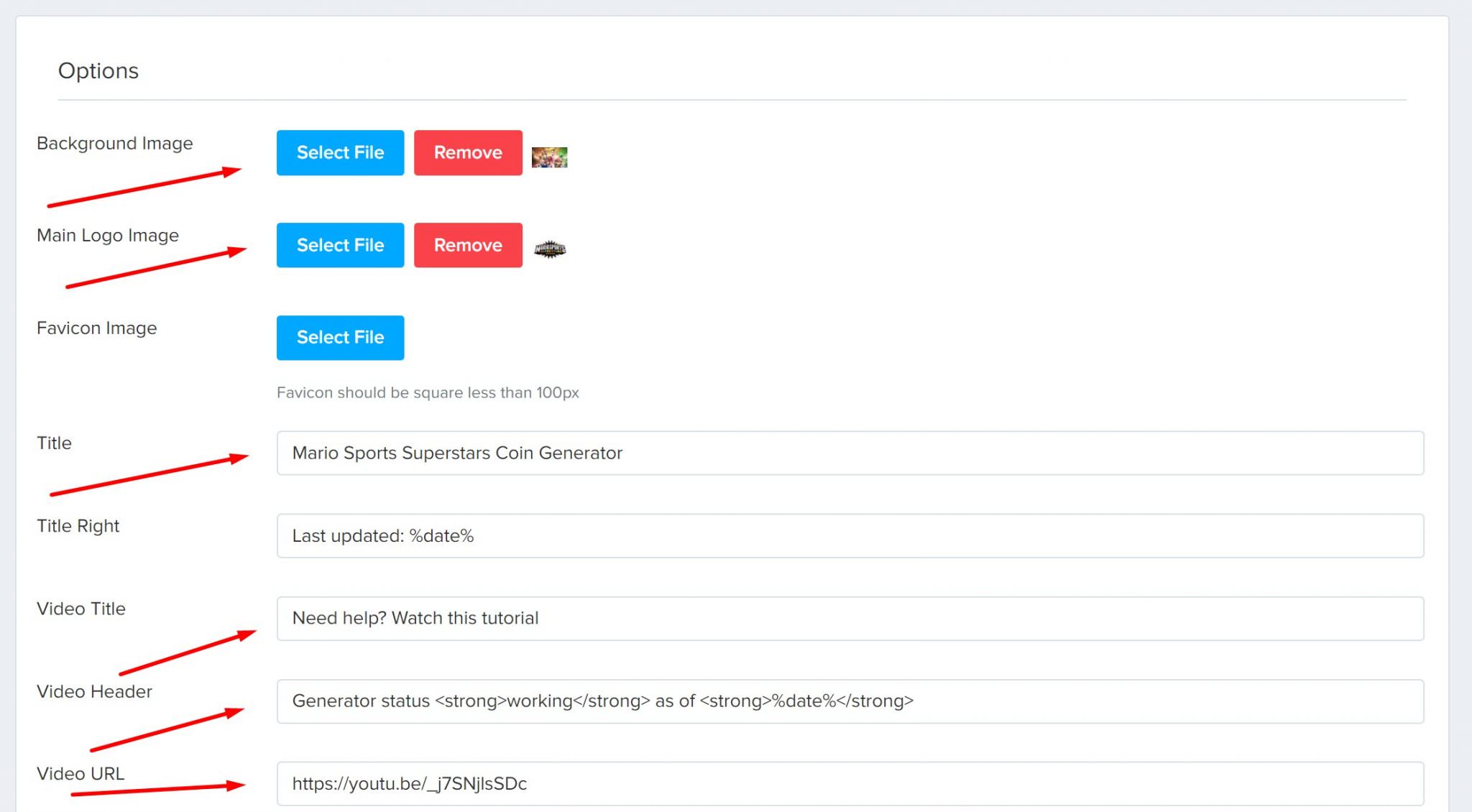**Options Page**

The image captures an options page with a clean white background. At the top left corner, the word "Options" is prominently displayed. The page is divided by a horizontal gray line which spans the width of the top section. Below this line, a series of customizable options is presented.

The customizable options include:

1. **Background Image**
2. **Main Logo Image**
3. **Favicon Image**
4. **Title**
5. **Title Right**
6. **Video Title**
7. **Video Header**
8. **Video URL**

Each of the first three options (Background Image, Main Logo Image, Favicon Image) features a blue "Select File" button to the right. Additionally, a red arrow points towards the "Select File" button for both the Background Image and Main Logo Image options. These two options also include a red "Remove" button accompanied by a small picture icon. Below the "Select File" button for the Favicon Image, a grey sentence reads: "Favicon should be square and less than 100px."

The remaining options (Title, Title Right, Video Title, Video Header, Video URL) each contain a text box with the following default values:

- **Title**: "Mario sports superstars coin generator"
- **Title Right**: "Last updated %day%"
- **Video Title**: "Need help? Watch this tutorial"
- **Video Header**: "Generator status: <strong>Working</strong> as of <strong>%date%</strong>"
- **Video URL**: "https://youtu.be/...J7SnJLSSDC"

Each of these text boxes is accompanied by a red arrow directing attention to the input fields to specify or edit the content.